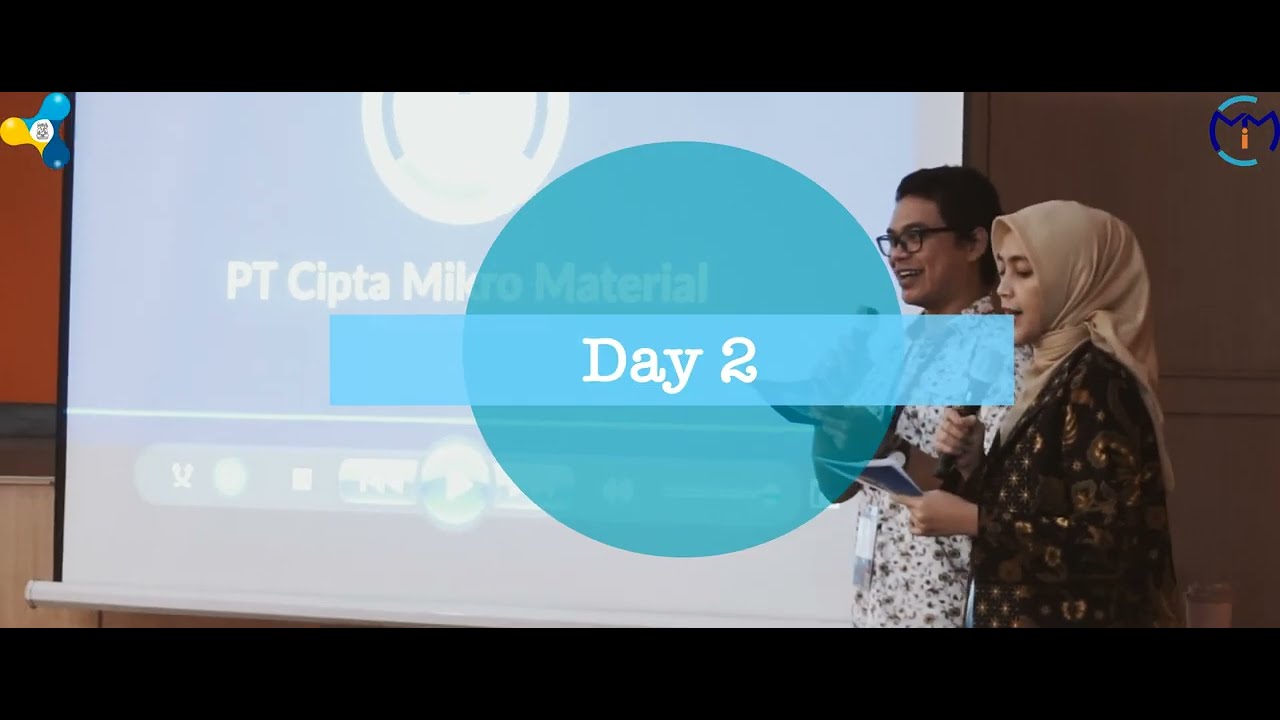In a conference setting, this photograph captures a detailed scene with a white projection screen prominently displayed at the center-back of the image, featuring the text "Day 2" in white font on a blue rectangular background. The screen also contains additional text, "PT Sipta Milk Crow material," accompanied by blue and yellow graphic elements, including a symbol resembling a fidget spinner on the left and a design that looks like a steering wheel with an orange "I" on the right.

Standing to the right of the screen, angled slightly to the left, are two individuals actively engaged in the conference. The man, positioned closer to the screen, has short black hair, wears glasses, and is dressed in a white shirt. He holds a microphone in his right hand and appears to be speaking. Next to him, a woman wearing a light brown headscarf and a dark brown coat adorned with white flower fragments is seen holding a brochure in her left hand and a microphone in her right, also seemingly in the midst of speaking. Both participants look to be about 30 years old, contributing to the dynamic atmosphere of the event.